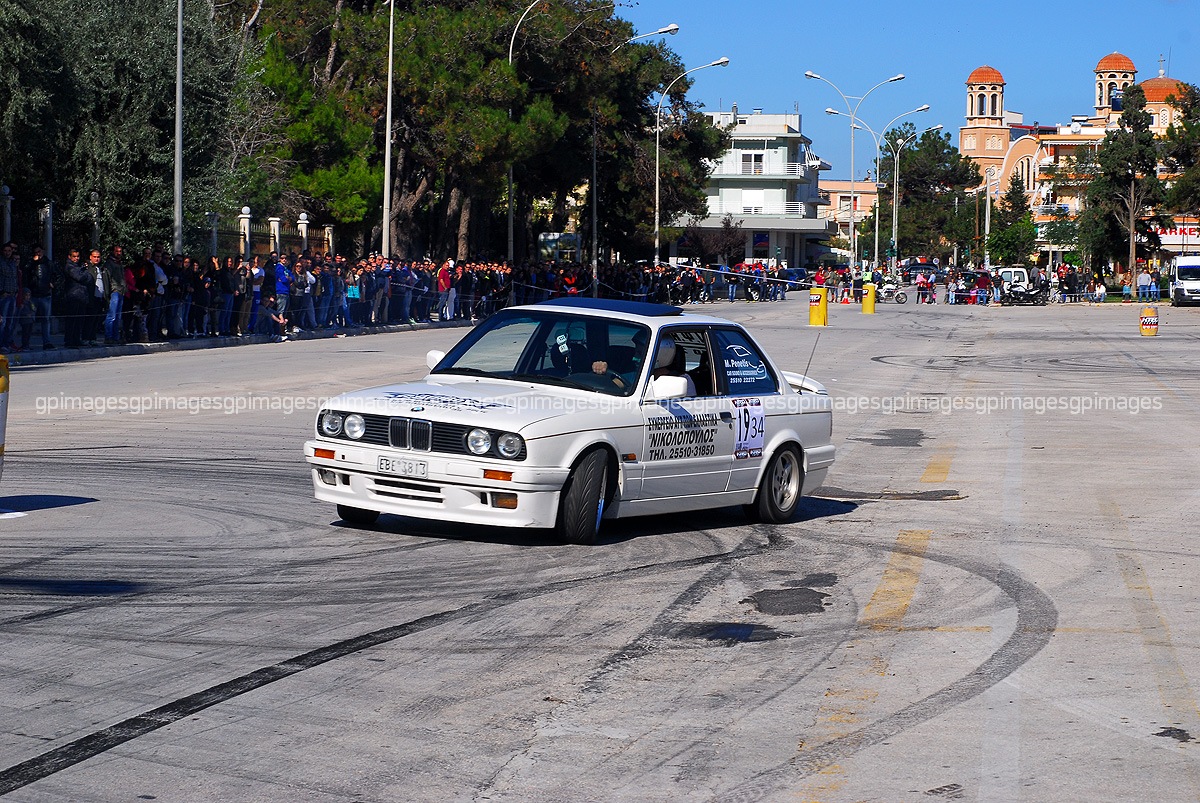This photograph captures a white, two-door BMW 3 Series, likely a 2+2 model, performing burnouts in the middle of an outdoor courtyard. The event is clearly a drifting or racing exhibition, with the car creating dramatic tire marks on the gray blacktop tarmac. The front wheels are turned sharply to the left, adding to the dynamic sense of movement. The BMW features black writing on the doors and hood, a white decal with text on the back window, and a notable racing number. The car includes distinctive elements such as two round headlights on each side and a chrome grille at the front. The sunroof is popped open, and the tinted passenger windows are also open. The driver inside is wearing a helmet for protection. Surrounding the car is a roped-off area ensuring safety, while spectators line the edges, standing on the sidewalk and behind light posts. In the background, there are tall green trees, several three- to four-story buildings, one of which resembles a church with an orange brick facade and a red tile roof. The entire scene underlines the thrill and community engagement in a regulated automotive event.